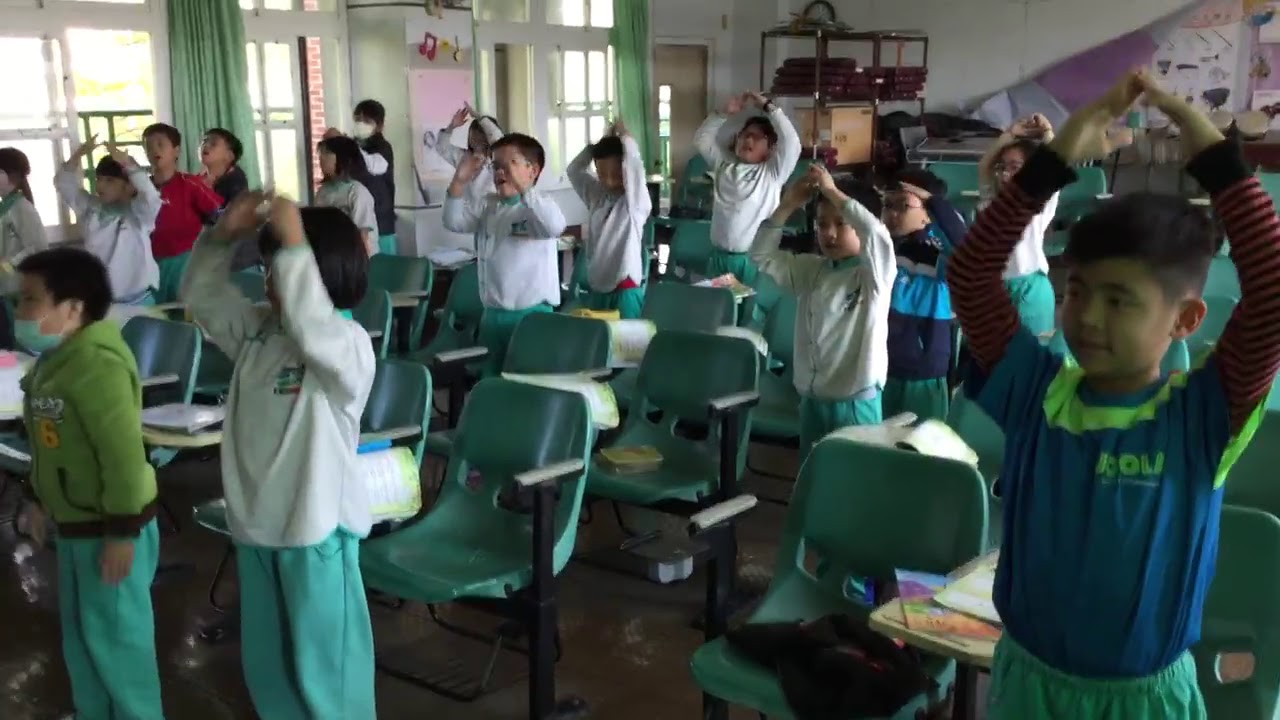This high-quality, vibrant photograph captures a moment inside an elementary school classroom. The image shows numerous children standing next to their unique conjoined desks, which feature green plastic chairs with black frames and a small wooden area in the middle, likely for resting books. The children, dressed in varied t-shirts but uniformly wearing light green or blue sweatpants, have their arms raised above their heads with their hands touching, possibly engaging in a stretching exercise or learning yoga. Some are seen wearing masks, while others are not, displaying a slice of the varied responses to health guidelines. Their expressions range from excited to confused, adding character and authenticity to the scene.

The classroom itself is well-lit with natural daylight streaming through undrawn light green curtains covering windows along one wall. These windows let in the bright daylight, enhancing the clarity and brightness of the image. The background is a mosaic of educational clutter, featuring shelves, boxes, and papers, along with a beige door edged with windows, providing a view into adjacent areas. In addition, a large portrait painting and some scattered posters add to the vibrant ambiance of the room. The overall setting is lively and dynamic, capturing the essence of a typical school day.